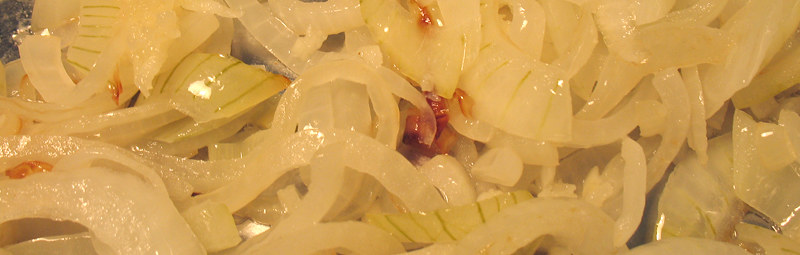This photo features a detailed, close-up shot of freshly fried onions. The image is in landscape mode, giving a clear view of the onions' glossy, slightly slimy texture, indicating they were fried in oil. The onions are mostly light yellow and whitish, with a few pieces having browned edges, suggesting they are in various stages of doneness. Some of the onions appear soft and tender, while others are slightly firmer. A notable detail is a single slice that is slightly greener, along with a hint of red in the middle of the image, possibly from an accidental splash of relish or ketchup. These onions, some diced and stringy, could easily be imagined as a topping for a hamburger or hot dog, adding to the overall appetizing appeal.